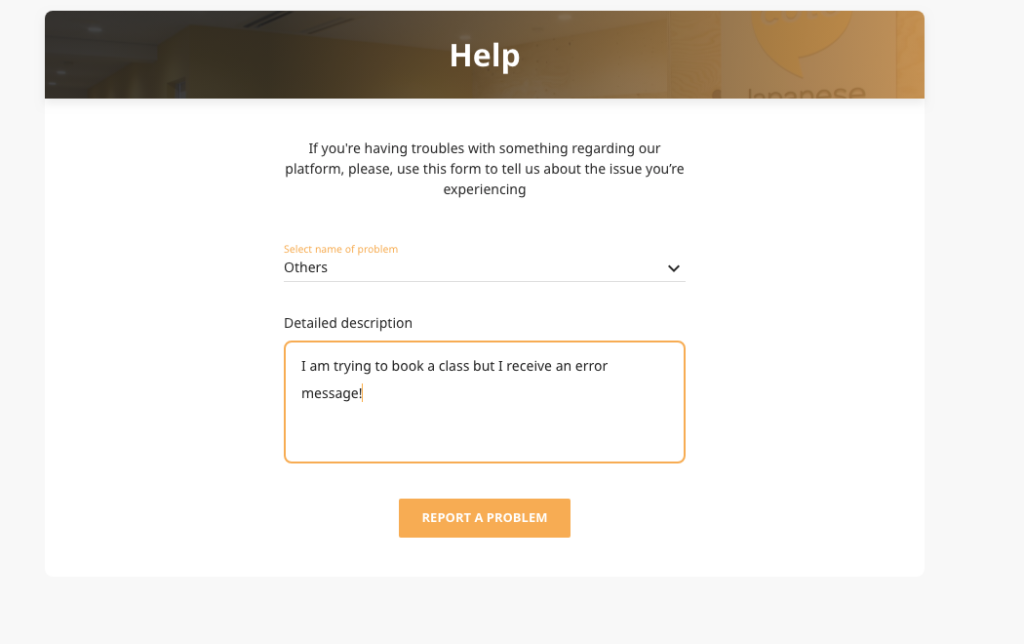The screenshot captures a HELP page from an institutional educational platform. The title bar, a muted black-brown hue, prominently displays the text "HELP" in bold. Centrally positioned, the word "HELP" is written in all caps. Beneath it, a message reads: "If you're having troubles with something regarding our platform, please use this form to tell us about the issue you're experiencing."

Further down, there's a dropdown menu labeled "Select name of problem," which currently shows "Others" as the selected option. Another section follows, titled "Detail description," featuring a white input box bordered by a yellow outline. This box contains the text: "I am trying to book a class, but I receive an error message!"

At the bottom of the form, a yellow button labeled "Report a problem" is visible. The overall background of this section is white, giving it a clean, approachable appearance.